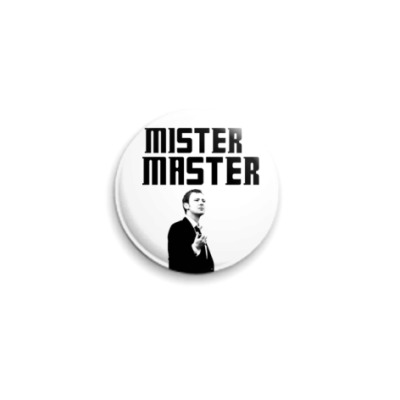The image features a close-up of a round, pin-back button set against a completely white background. The button itself has a white base and prominently displays black text at the top, arranged in two rows. The first row reads "Mr." and the second row reads "Master," both in bold, left-justified, futuristic font. Notably, the "S" characters in both words resemble the number "5," with sharp edges, and the "I" in "Mr." as well as the "M" in both "Mr." and "Master" have edges that slightly tilt to the left.

Beneath the text is a high-contrast, black-and-white photograph that has been filtered to appear as line art. The photograph depicts a clean-shaven Caucasian man with dark hair, wearing a black suit, white-collared dress shirt, and a tie. The man is shown from the top of his head to about his waist, standing at a three-quarter angle and facing right. His right arm is bent at the elbow, with his forearm and hand raised to the height of his clavicle, appearing as if he is speaking or gesticulating. The man's gaze is directed slightly upwards. There is a slight shadow cast at the lower left rim of the button, adding depth to the otherwise flat, graphic representation.